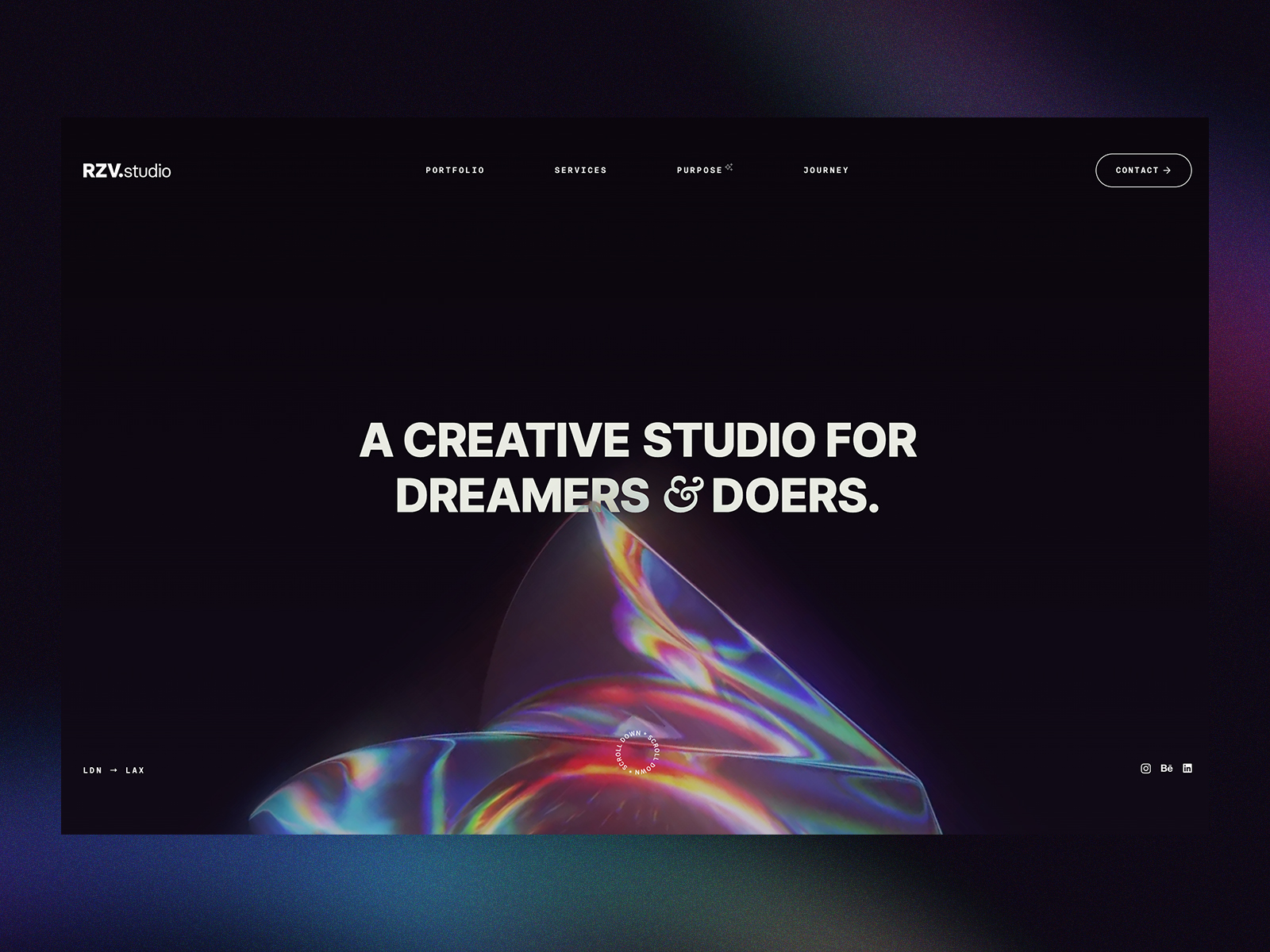The image is slightly wider than it is tall, roughly by about 20%. The background features a smooth, blurred gradient transitioning from black in the upper left, through purple towards the right, and finally into blue as it moves downward. Overlaid on this gradient is a website interface, occupying around 80% of the image space. 

In the upper left corner of the website, against a black background, white text reads "RZV" in bold capital letters, followed by ".studio" in regular font. Moving towards the center, a navigation menu is visible with the options: Portfolio, Services, Purpose, and Journey. On the right side of the menu, there is a black button outlined in white with the word "Contact" in white lettering.

Dominating the center of the image, in large bold capital letters, is the phrase "A CREATIVE STUDIO FOR DREAMERS AND DOERS." At the bottom of the image is an abstract piece of art with an oil-like color pattern. This piece resembles a surfboard, oriented to the left, with a shark fin-like shape on top. The lower half of the surfboard is cut off, adding to the artwork's unique and obscure aesthetic.